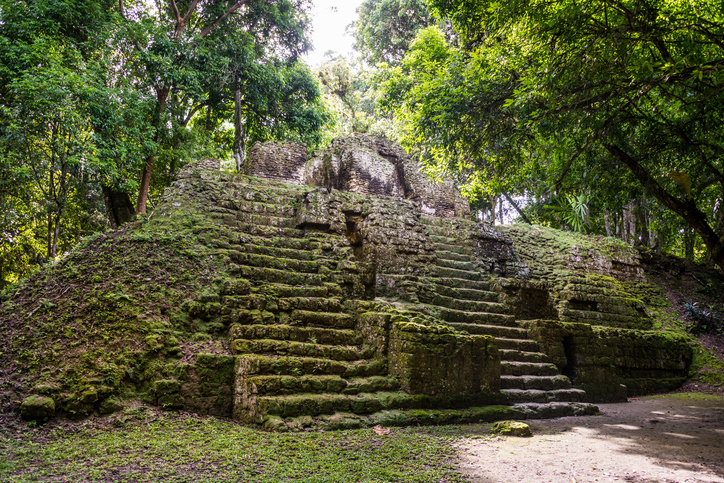The photograph depicts an ancient temple, likely part of Mayan, Incan, or Aztec ruins, situated in a dense Latin American rainforest, possibly Mexico. The stone structure is composed of old, weathered gray rocks, prominently covered in green moss, adding to its ancient and mystical appearance. The temple ruins are positioned diagonally from the left middle to the right middle of the image, with broad stone steps leading up to a higher platform. The steps themselves are wide and partially obscured by moss and square block stones. Surrounding this historical edifice are lush trees with varying shades of green leaves, including bright lime and forest greens. The ground is covered with grass and casts heavy shadows interspersed with beams of sunlight filtering through the canopy. The entire scene is bathed in natural daylight, enhancing the stone's textures and the vivid green foliage of the surrounding jungle. The setting captures the essence of a timeworn sanctuary enveloped in nature’s embrace.